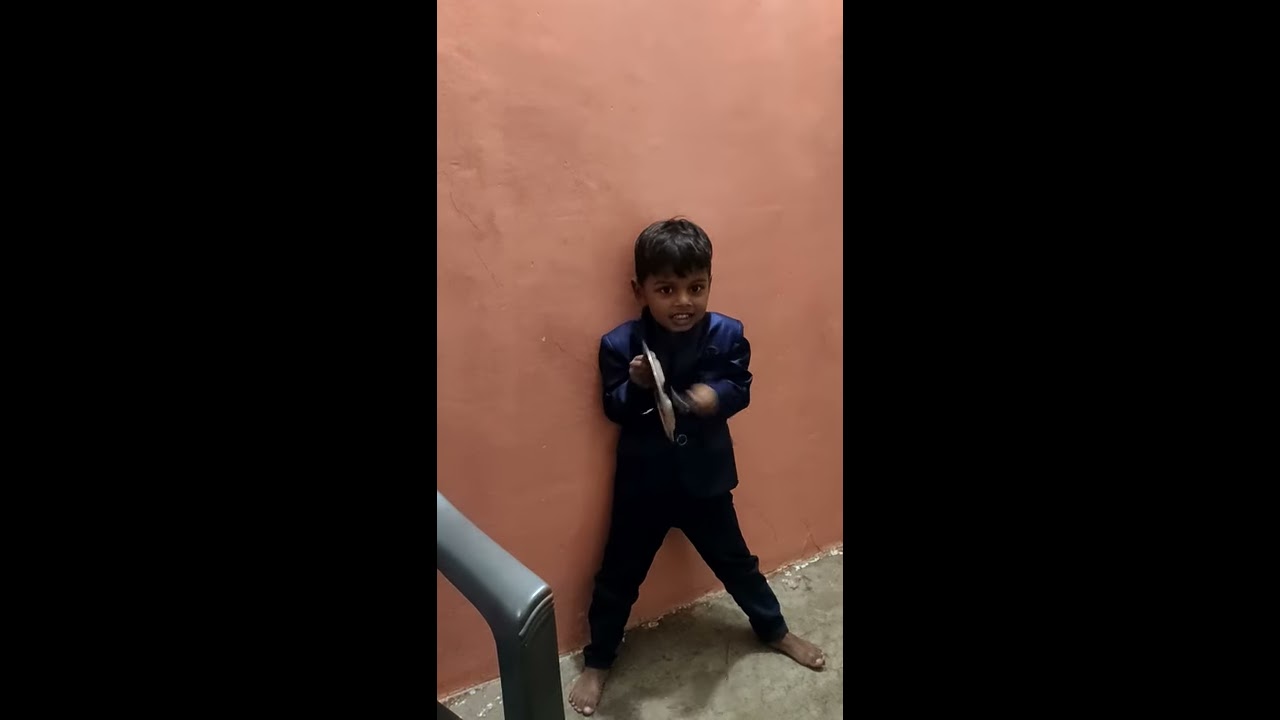In the image, a young boy stands barefoot on a concrete ground, against a light orange, slightly rough wall reminiscent of adobe. He has brown skin, black hair just above his eyebrows, and expressive brown eyes. The boy, dressed in a blue long-sleeve shirt resembling a dress jacket and black pants, seems to be mid-motion with his arms creating a swishing blur. His legs are spread apart, indicating a dynamic stance. He holds an indeterminate object close to him—it could be sunglasses or a plate being tapped with his other hand. A faint shadow is cast by him against the wall and on the ground. In the lower left corner, part of a metal chair is visible, adding to the scene's nuanced detail.